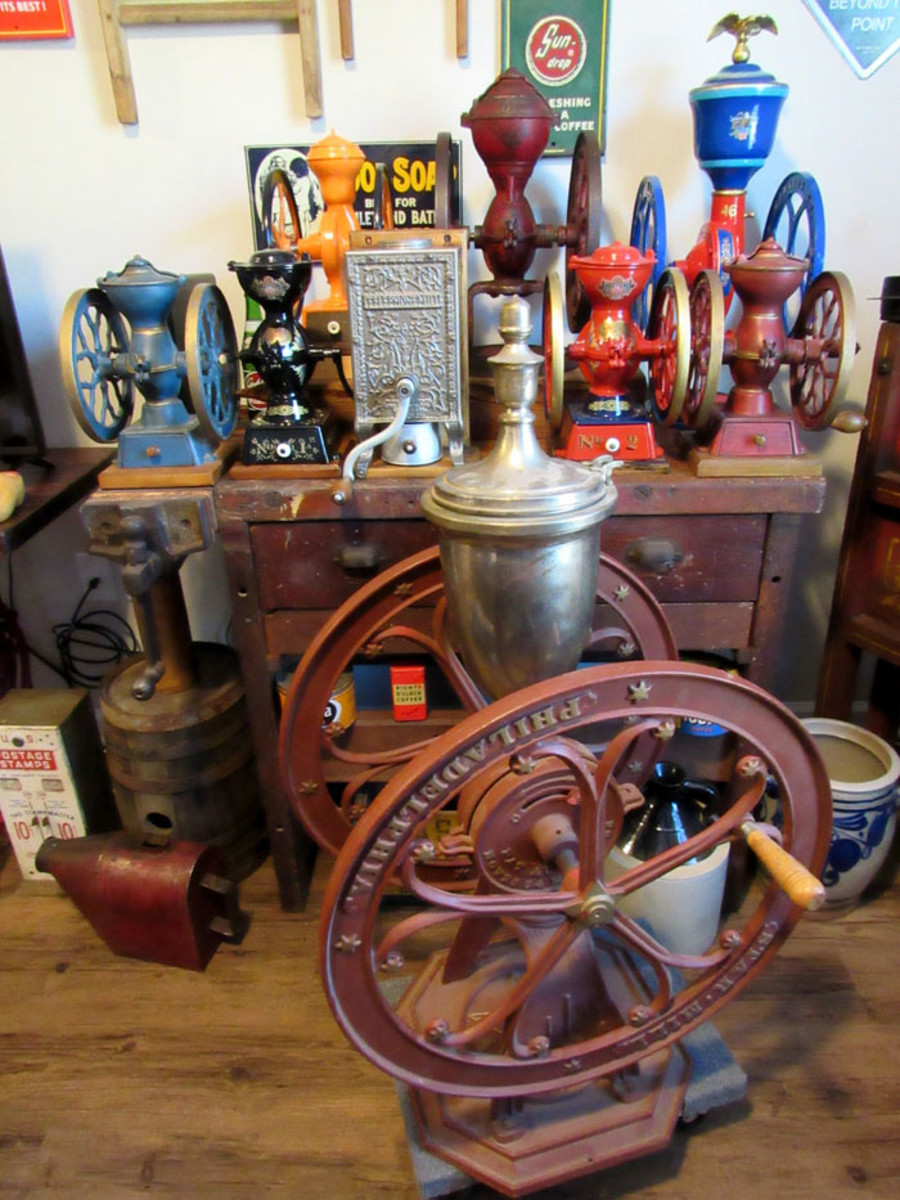The photograph captures a room filled with an intriguing collection of antique mechanisms, prominently featuring various hand-crank-operated devices. The room has a wooden floor and a white wall at the far end, adorned with several vintage tin signs. Dominating the back of the room is a sturdy brown wooden cabinet displaying numerous gear-like and crank mechanisms, meticulously arranged. In front of this cabinet sits a large gear mechanism on the floor, distinct in its size and placement.

Among the collection, there are numerous colorful cranks, each with its unique attributes. The frontmost crank has a silver cup on top, flanked by two wheels with wooden dowel handles, and bears the faded inscription "Philadelphia Mill." These devices are likely used to grind grains, possibly for coffee. The collection includes cranks of various colors: blue, black, silver (mounted on a box with a front-facing crank), orange, red, darker red, and a combination of red and blue. These historical hand tools rest on weathered, antique-looking furniture, adding to the room's nostalgic ambiance.